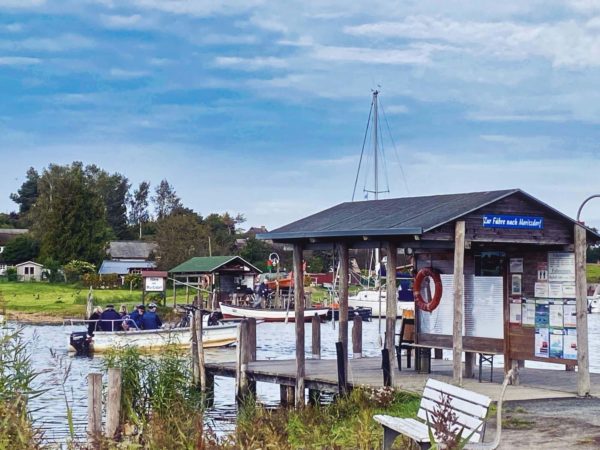This color photograph captures a serene boating area under a light blue sky with thin, wispy clouds. Dominating the right side of the image is a small pier constructed out of wood, featuring a great triangular rooftop supported by several wooden pylons. Underneath this roof on the wooden brown floor of the pier, there is a brown bench. The right side of the pier has a wooden wall adorned with a blue sign with white writing at the top, various sheets of paper, photographs, a red life preserver, and a billboard. In front of the pier, a yellow or beige motorboat, complete with a silver front fence and a black motor, is filled with people wearing blue life jackets. This boat is situated on a tranquil river surrounded by vegetation, which includes tall grass in the foreground. Behind this boat, another covered pier with a green roof and occupied by a red and white boat is visible on the opposite shore. The surroundings feature green trees, a small field, and additional structures such as outbuildings or barns, creating an overall picturesque and lively scene.